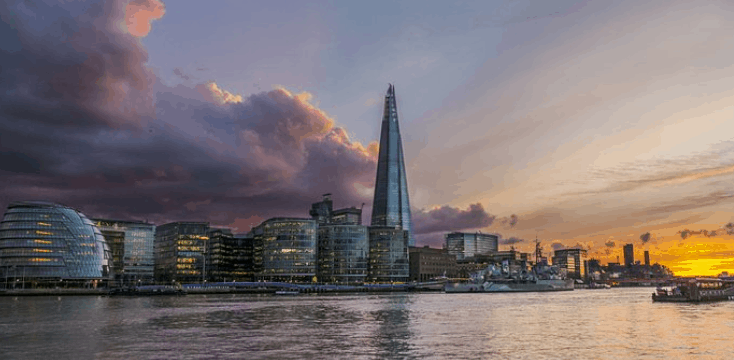The image captures a stunning city skyline at dusk. A large body of water occupies the bottom, reflecting the skyscrapers and a small squat longboat moving from left to right. The centerpiece of the skyline is a towering, triangular-shaped building known as the Shard, flanked by multi-story buildings on both sides. The leftmost structure is distinguished by its dome-shaped top. The scene is marked by a range of colors including blue, gray, purple, pink, yellow, and orange. Thick, gray, rain-laden clouds hover in the top left of the sky, juxtaposed against the lighter blue sky and a beautiful yellow-orange sunset to the right. The overall cityscape has a modern, clean appearance, with some buildings subtly lit, suggesting urban vibrancy transitioning into night.